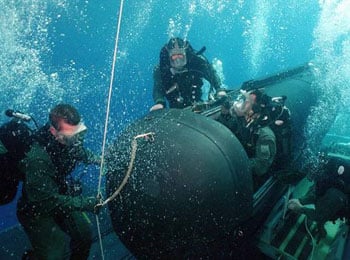In the photograph, four scuba divers are submerged underwater, fully equipped with scuba gear, including masks, tanks, and diving suits. They are working on a sleek, black, bullet-shaped submersible vehicle with an open hatch. The vehicle is situated predominantly in the bottom right corner of the image. One diver is seated inside the submersible, adjusting controls or components, while another diver stands directly opposite him, holding onto the vehicle and observing the work being done.

To the far left, another diver is positioned in front of the submersible, examining the equipment and holding onto a cable or hose connected to it. This diver also steadies a long rope or hose extending vertically through the water. In the bottom right corner, a partially obscured fourth diver appears to be inspecting or repairing another part of the submersible, possibly situated on a platform.

The scene is enveloped in a vivid blue hue of underwater light, with bubbles streaming upwards from the divers, indicating their continuous breaths and adding dynamic texture to the aquatic environment.